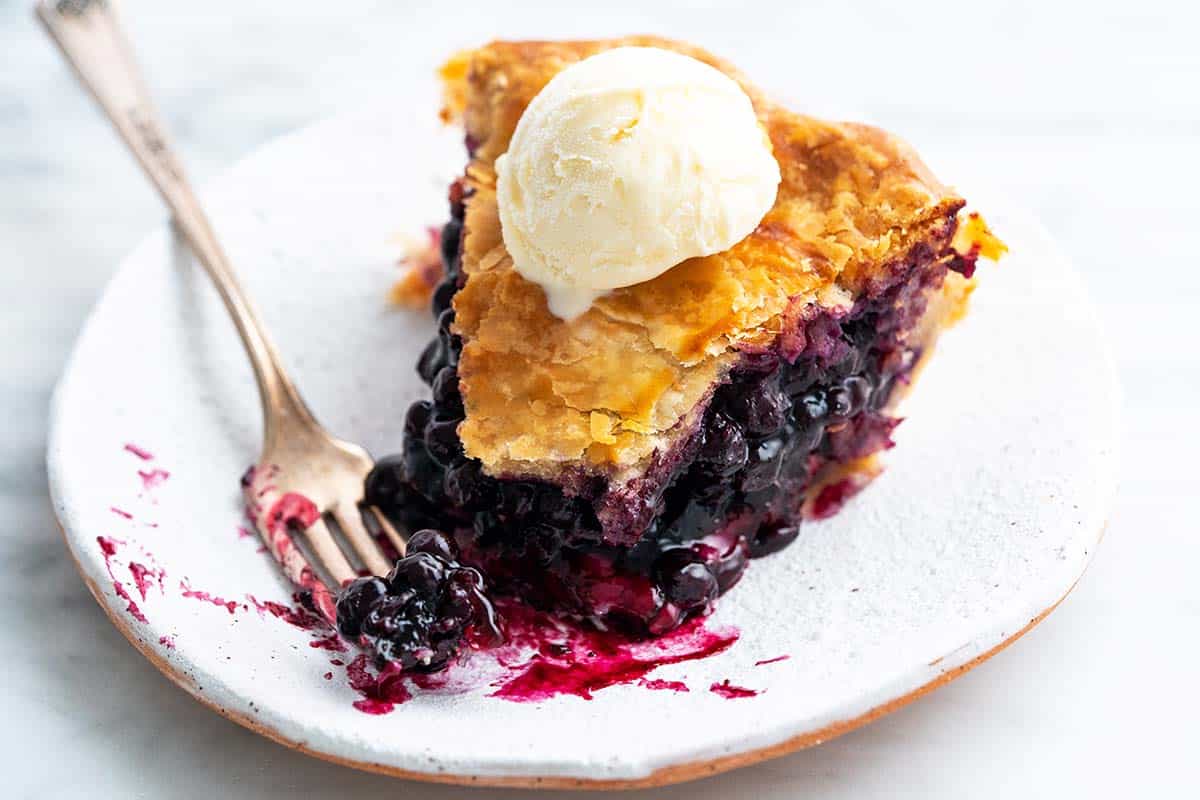A sumptuous slice of blueberry pie rests on a white clay plate with a brown underside, set on a white table. The pie, brimming with dark purple, juicy blueberries, features a golden, flaky crust. A perfectly round scoop of vanilla ice cream crowns the pie, just beginning to melt, with a droplet cascading down onto the crust. To the left, a silver fork, streaked with blue and adorned with a couple of blueberries, suggests a bite has been taken. Bright magenta-purple juice from the pie adds a vivid splash of color on the plate. This dessert scene exudes an inviting, mouthwatering allure.